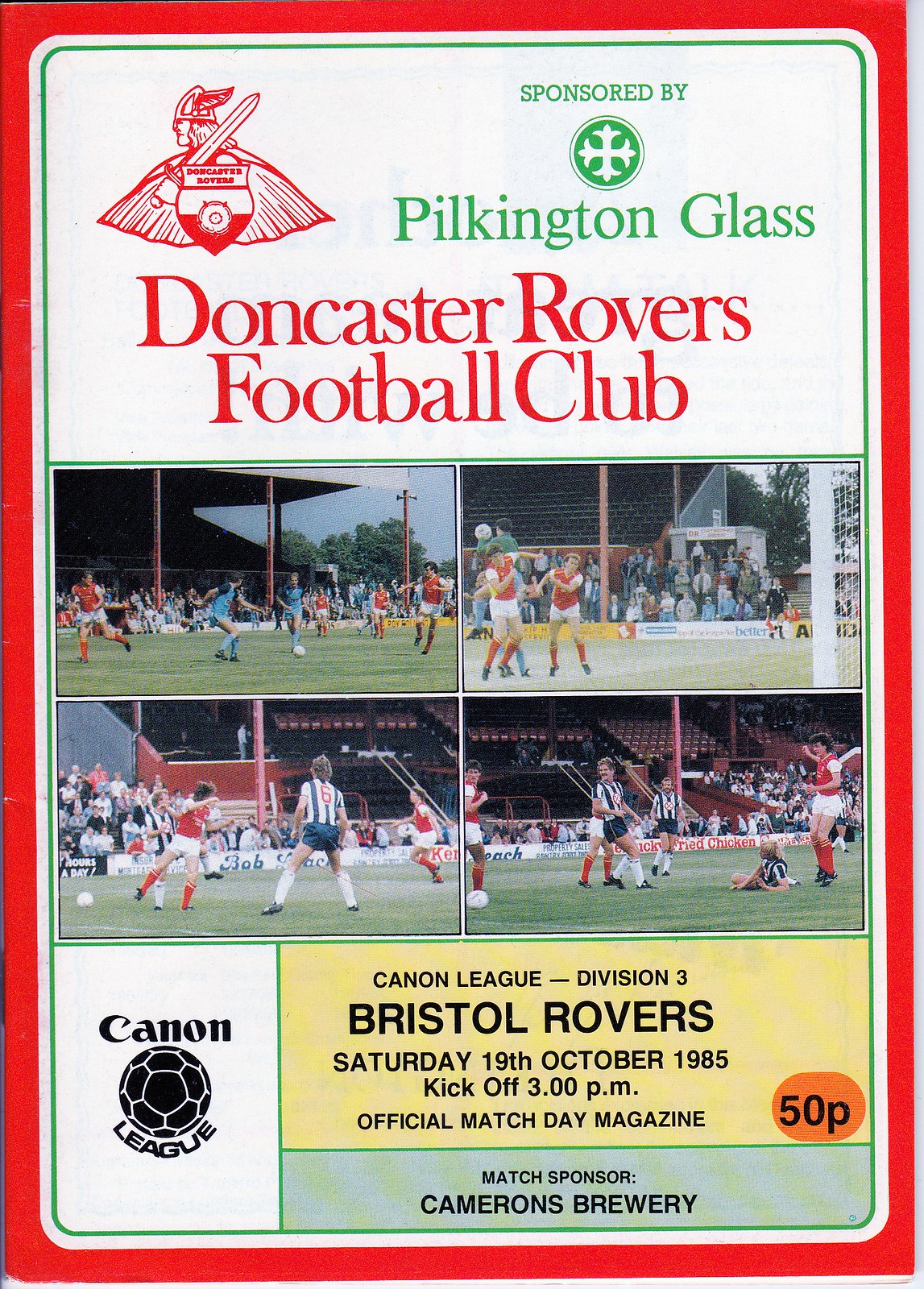This cover of a football program from October 19th, 1985, is a nostalgic piece from a match between Doncaster Rovers Football Club and Bristol Rovers in the Cannon League Division III. Sponsored by Plankington Glass, the white and red theme prominently features the Doncaster Rovers insignia—a Viking wielding a sword—at the top. Four color photographs capturing action shots from a match are positioned at the center, with one on each corner. Beneath these images, in a yellow section, pertinent details are displayed: "Cannon League Division III, Bristol Rovers, Saturday, 19th October 1985, kickoff at 3 p.m., Official Match Day Magazine." A small orange sticker indicates the price, "50P." Lastly, the bottom section includes the match sponsor, Cameron's Brewery, and a green Cannon League logo featuring a soccer ball, confirming Cannon's sponsorship of the event.